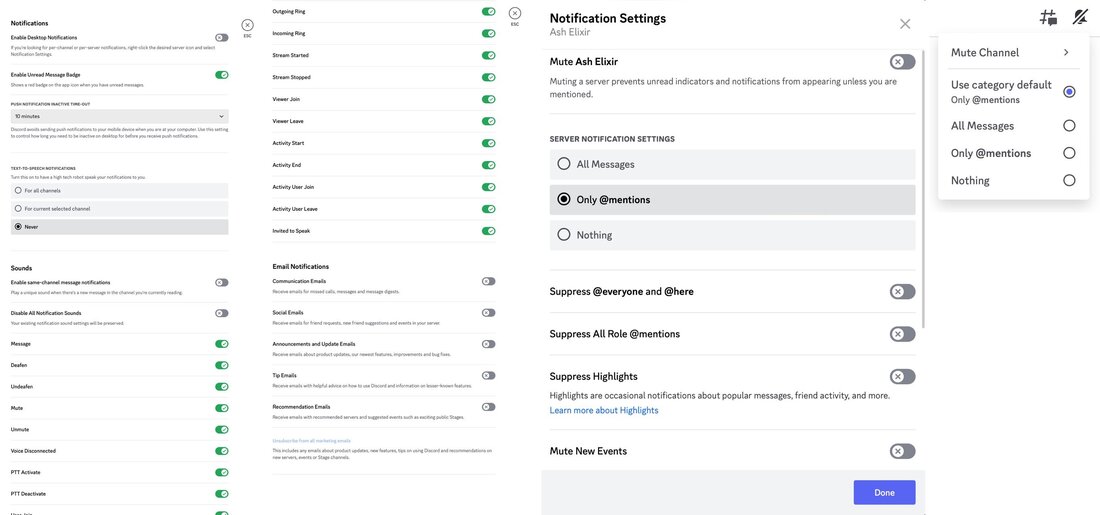This image showcases a collection of screen captures, depicting several notification windows from a user interface. The screen captures are arranged in three or four columns. The farthest column on the left features a notification window, which includes a descending list of information accompanied by slider buttons at the bottom. The text is not clearly legible due to the image's fine resolution.

To the right of this first column, there is what appears to be a continuation of the information, where detailed descriptions are visible on the left. Adjacent to each description on the right are green slider buttons, indicating active settings.

Towards the center-right, there is another notification setting screen, larger and more readable. This window contains text that reads, "Mute ASHELIXIR." Below this, there is a description explaining that muting the server prevents unread indicators and notifications from appearing, unless the user is directly mentioned. Further down, there is a section labeled "Server Notification Settings," featuring options such as "All Messages," "Only Mentions," and "Nothing." Additionally, there are three lines of settings with unselected slider buttons. These settings include options to "Suppress @everyone," "Suppress All Role," among others.

Overall, the image details various notification settings and options, demonstrating how users can customize their notification preferences within the interface.